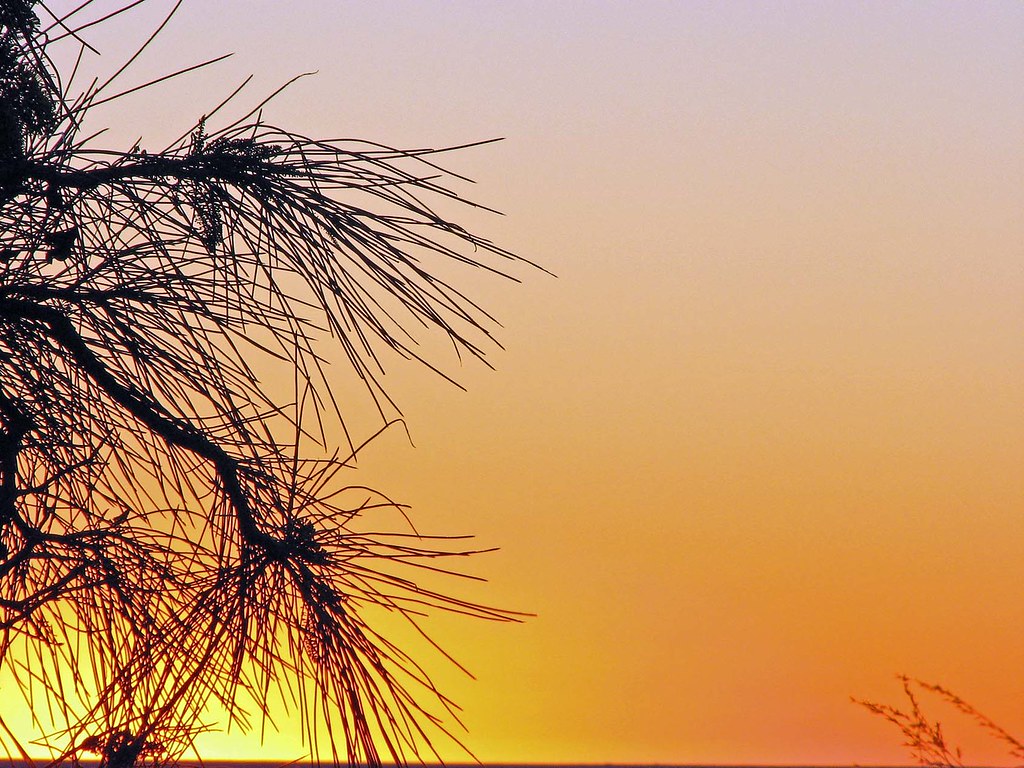The photograph captures a breathtaking sunset, where vibrant colors blend seamlessly across the sky. At the bottom of the image, a radiant yellow sun emerges over the horizon, gradually transitioning into a warm turmeric yellow that extends towards the right side. This hue deepens into a rich burnt orange, which envelops the sky around the sun. Higher up, the sky transitions into a soft pink, blending into a light purple, culminating in a deep, dark purple at the top of the image. Silhouetted in black against this gradient of sunset colors are three branches adorned with long, thin clusters of pine needles, providing a striking contrast to the vivid sky. Additionally, a small plant peeks into the frame from the bottom right corner, subtly accentuating the dynamic interplay of natural elements within the scene.